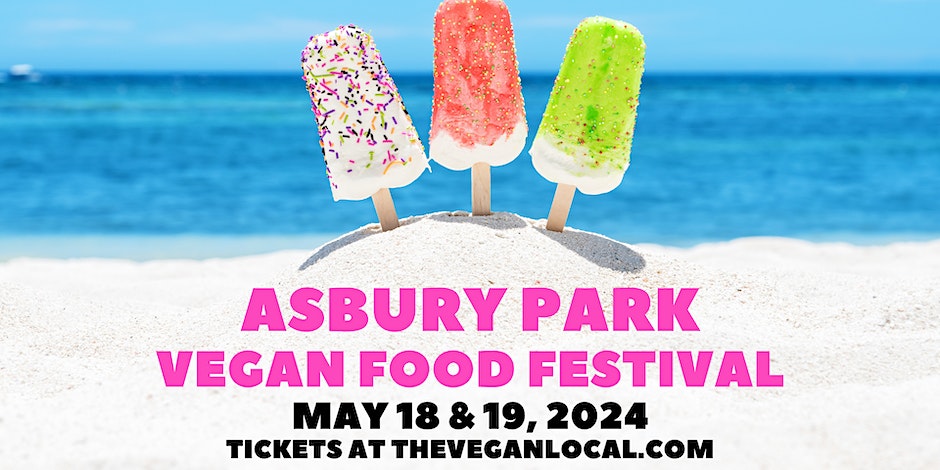The image is a horizontally oblong advertisement for the Asbury Park Vegan Food Festival, set for May 18 and 19, 2024, in New Jersey. The top half features a serene scene of a light blue sky meeting the ocean, with a faded image of a small white boat visible in the upper left corner between sky and water. Transitioning downward, the image showcases bright white sand forming a central dome. Positioned on this mound of sand are three popsicles. 

The popsicle on the left appears to be vanilla with an array of pink, purple, green, red, and orange sprinkles. The middle popsicle also looks vanilla-based but features a bright orange coating with sprinkles of yellow and green. The popsicle on the right has a light green, possibly lime-flavored coating with red, orange, and yellow sprinkles. 

Beneath this vibrant scene, in bold raspberry-colored print, the text reads, "ASBURY PARK VEGAN FOOD FESTIVAL." Below this, in bold black text, it announces the dates, "May 18 and 19, 2024." The final line, also in bold black but smaller print, provides ticket information: "Tickets at theveganlocal.com."